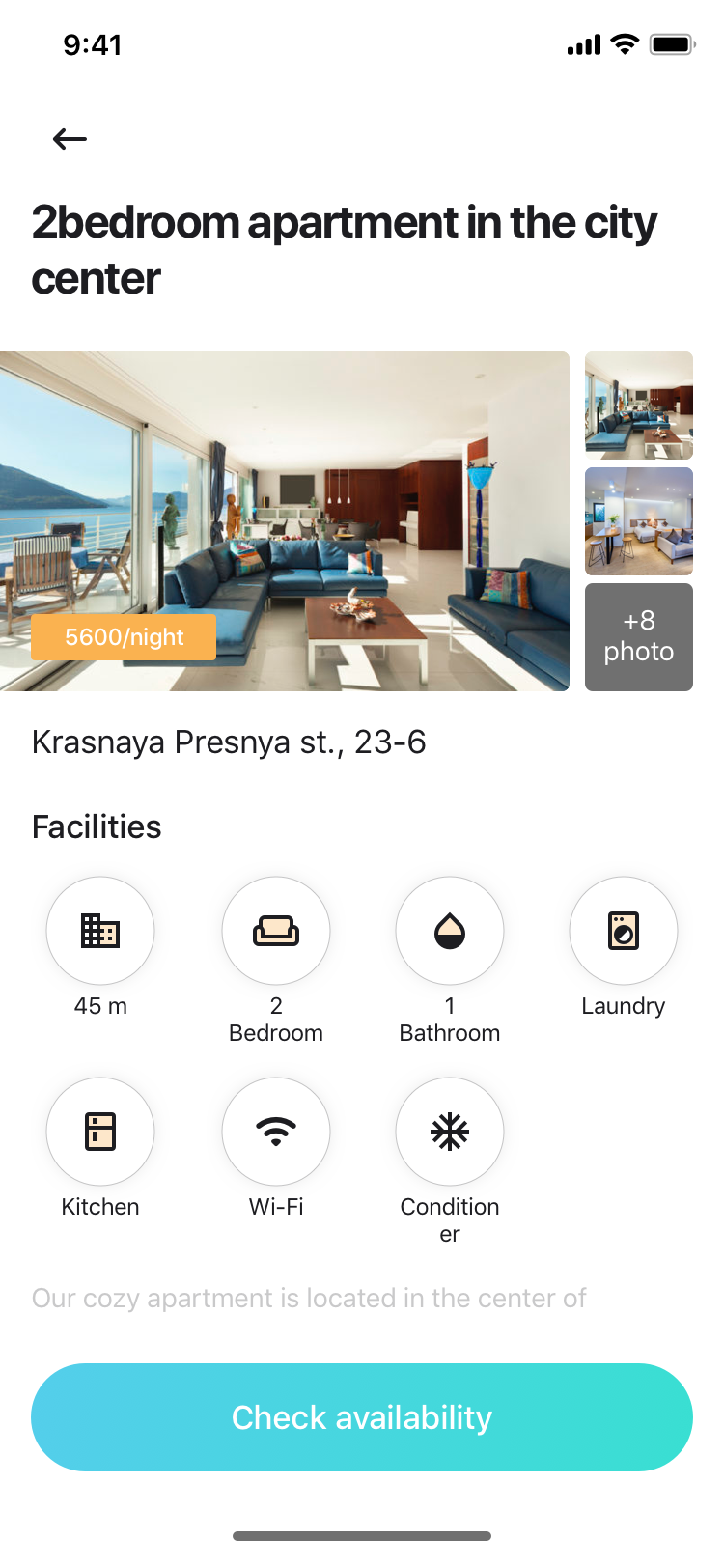A vertical image displays what appears to be a screenshot of a smartphone, either an Android or iPhone, showcasing an apartment listing. At the top, the status bar displays typical elements: "941," signal bars, Wi-Fi symbol, and a full battery icon. Below, a black left-pointing arrow and text reading "Two-bedroom apartment in the city" introduce the listing.

The main image is a long, rectangular photo of a luxurious apartment. It features teal sofas, a central wooden table, white floors, and a white ceiling. In the background, a kitchen with wooden cabinets is visible. Through the window, a scenic seascape with a hillside and beach chairs can be seen. To the right, there are a few small, stacked nature photos, though their details are unclear. Below the main image is a gray box with white text indicating "+8 photos."

Under the photos, the address "Krasnaya ST 23-6" is listed, along with the apartment's amenities: "Facilities, 45 minutes to town, Two-bedroom, one-bathroom, laundry, kitchen, Wi-Fi, air conditioning." Further details about the apartment are partially obscured with faint gray text that begins, "Our cozy apartment is located in the center of..."

At the bottom, there's a teal "Check Availability" button, along with a gray bar. An orange box on the main apartment image indicates the rate, "5600/night," in white letters. The address "Krasnaya ST" suggests an Eastern European location, likely in Russia.